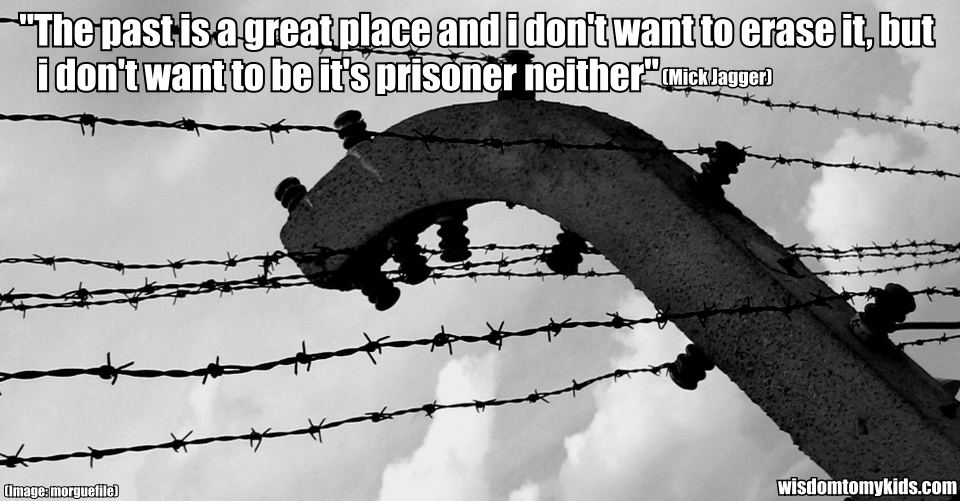This black-and-white photograph depicts a stark barbed wire fence stretching across a cloudy gray sky. The main feature is a slightly curved, dark metal post adorned with twisted, coiled ceramic holders to which the barbed wire is attached. Seven distinct rows of barbed wire, each lined with sharp spikes, run horizontally across the image, cutting through the bleak sky. 

At the top of the photograph, a poignant quote by Mick Jagger is prominently displayed in white text against a black border: "The past is a great place and I don't want to erase it, but I don't want to be its prisoner either." Mick Jagger’s name appears in small font within parentheses, following the quote. Additional text credits "Image Moogfelt" in the lower left corner and "wisdomtomykids.com" in the lower right corner, adding to the context of the visual message conveyed by the photograph.